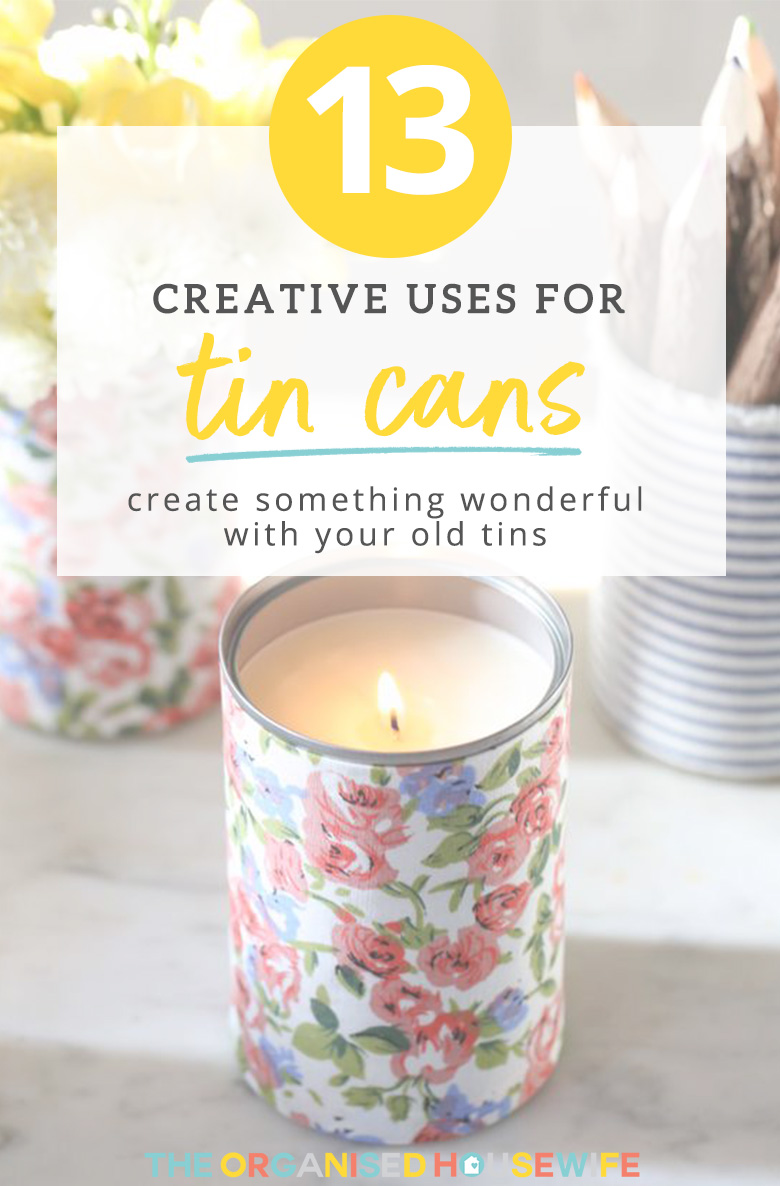A cozy, inspiring header image perfect for a personal blog or lifestyle website, featuring a collection of stylishly repurposed tin cans. At the forefront, a plain white candle burns warmly inside a tin can wrapped in beautiful floral fabric boasting pink, blue, and green hues. Behind it, another can with the same floral pattern serves as a charming vase for fresh flowers, while a third can, adorned with a blue and white striped design, holds a myriad of colored pencils. All of these are artistically arranged on a sleek marble countertop. The text overlay reads "13 Creative Uses for Tin Cans" in bold white letters inside a yellow bubble, followed by "Create Something Wonderful with Your Old Tins" in cursive, underlined in blue. At the bottom, the vibrant multicolored logo of "The Organized Housewife" ties the image together, hinting at a creative and organized lifestyle.